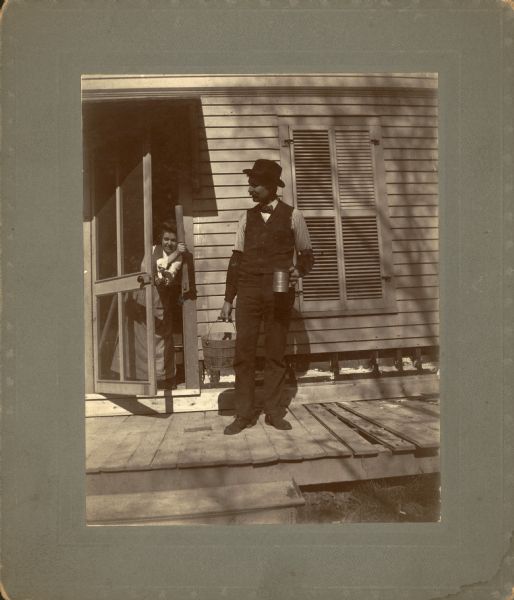The black and white photograph, reminiscent of an earlier era, is framed with a thick gray border, capturing a vintage moment in time. Taken in portrait orientation, the image depicts the side of a house that evokes the essence of Amish country. Central to the composition is a man who bears a striking resemblance to Charlie Chaplin, complete with a mustache and his iconic attire: a black top hat, a bow tie, a dark vest, black slacks, and black shoes over a long-sleeve white shirt. He dons dark armbands on his sleeves and holds a tin mug in his right hand and a wooden bucket in his left. Standing on a wooden boardwalk-style porch, he looks off to the left with a contemplative expression. To his left, a woman emerges from a partially open screen door, her head peeking out. She wears traditional Amish-style clothing, comprising a long dark dress with a white blouse underneath. The woman’s presence is subtle yet noticeable as she holds a wooden stick or rolling pin. Behind the man, a slatted window adds to the rustic charm, while the porch itself shows signs of wear with a few holes near the edge, reinforcing the photograph's antiquity.